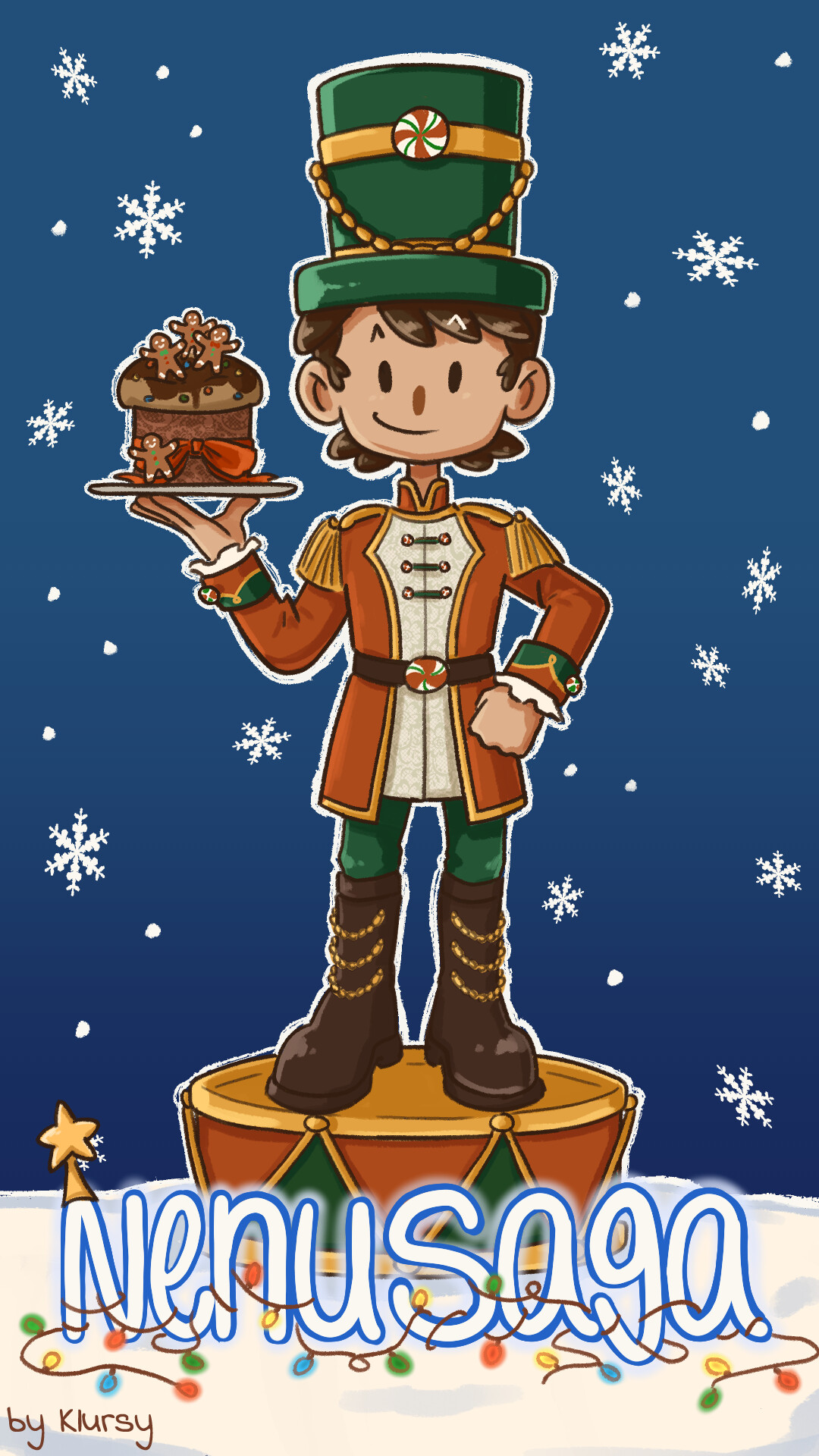The image depicts a cutesy, cartoonish-style illustration reminiscent of a greeting card. A figure resembling a toy soldier or nutcracker takes center stage, standing atop a golden-brown drum adorned with green and gold triangle patterns around its edges, set against a blue background with falling snowflakes. The character wears a green top hat featuring a peppermint candy at its center and a gold ribbon wrapped around the hat, accentuated with golden rope towards the top. He has simplistic, round eyes with a dot-smile face and brown hair.

He is dressed in an orange-red marching band jacket with gold shoulder pads and frills, green cufflinks with peppermint symbols, and an inner vest held together by pins that also have peppermint motifs and green ribbons. His ensemble includes green pants and brown shoes with three golden laces each. He sports a peppermint candy belt buckle.

In his left hand, he holds a decorative cake on a gray platter. The cake is adorned with three gingerbread men, two of whom wear green ties with red buttons, while the third has a red tie and green buttons. The cake, with brown icing and a red ribbon, is intricately detailed with embroidered designs.

The scene is festive with the text "Nunasanga" outlined in blue, topped with a party hat with a star, and illuminated by intertwined Christmas lights in green, yellow, red, and blue. The artist's name, Klersy, is signed at the bottom left in brown. The overall aesthetic is cute and whimsical, perfect for a holiday greeting.